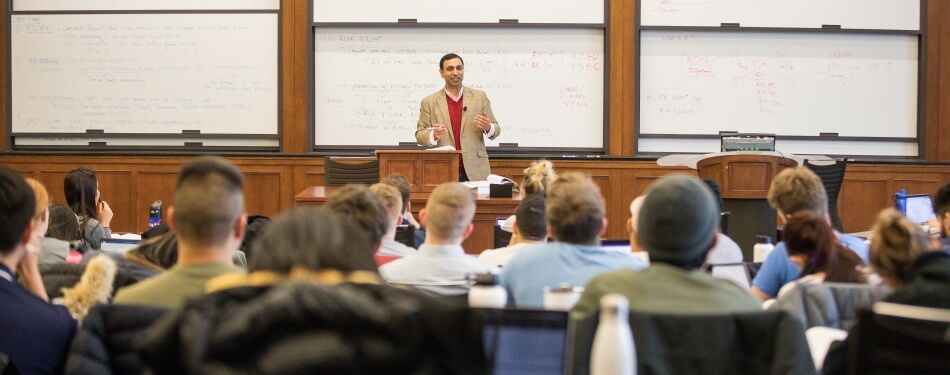The image captures a seminar or meeting inside a boardroom or classroom. A man with brown hair, wearing a tan blazer over a red shirt, stands behind a wooden lectern at the center, addressing a seated audience. His hands are raised as he speaks, engaging with the listeners. The backdrop consists of three large whiteboards filled with multicolored writings, predominantly in reds and greens, covering the entire background. Around 15 people are seated, facing away from the camera, their varied hairstyles and clothing visible. Notably, a man in the foreground, slightly left of center, sports a light green shirt and a military-style short haircut. Another individual, to the right, wears a gray beanie and a green shirt. A woman seated towards the front row has brunette hair and holds her right hand to her face. An unidentified white object, possibly a bottle, is visible at the bottom right of the image. The overall scene depicts an attentive audience immersed in the session led by the dynamic speaker.